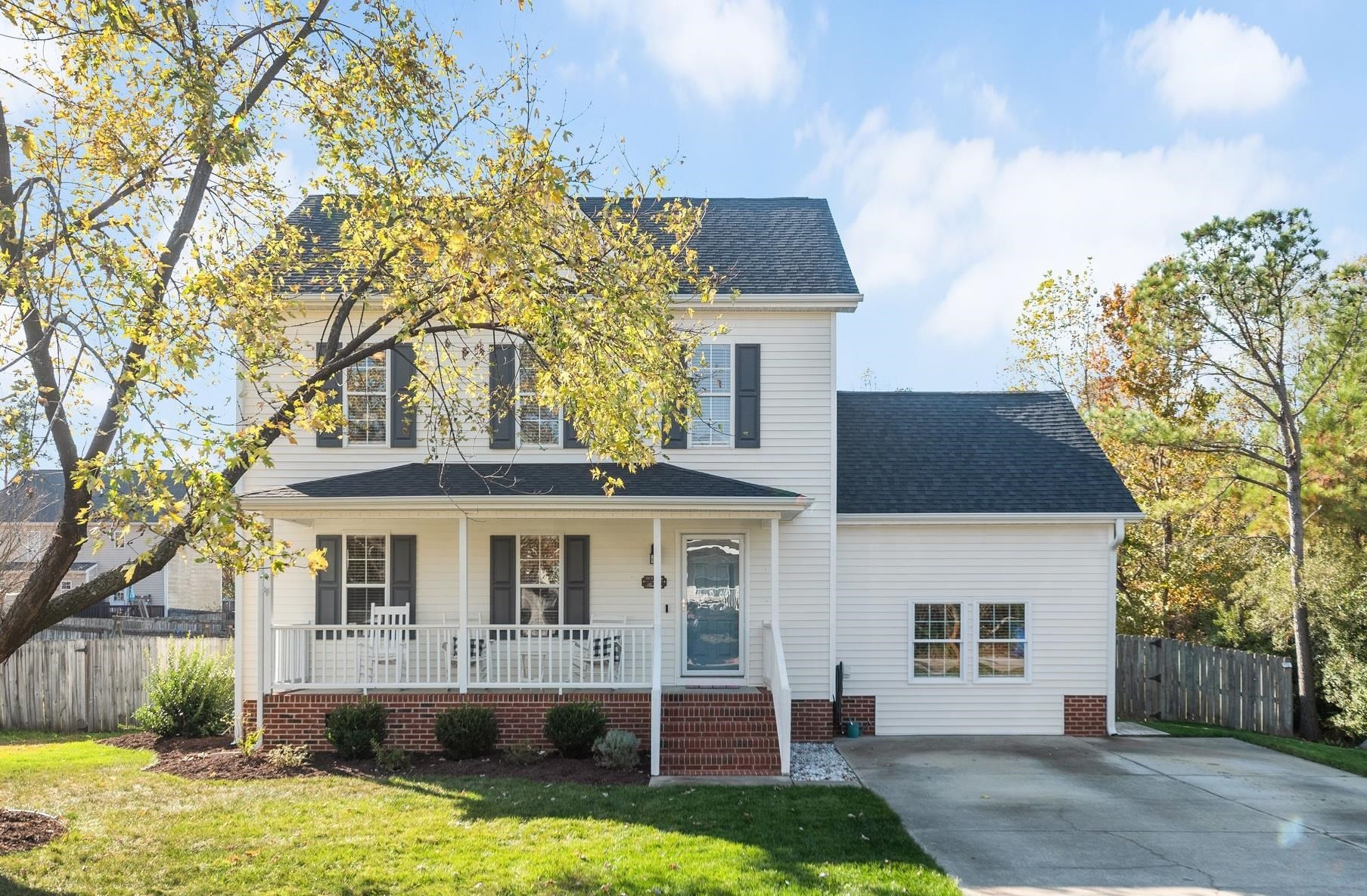The image depicts a traditional, colonial-style countryside home with white paneling and a gray, gabled shingle roof. The two-story rectangular structure has five shuttered windows, three on the second floor and two on the first, flanking a blue door with a clear glass storm door. The front porch, featuring three white rocking chairs, is supported by four columns and enclosed by a white picket fence, with a brick staircase leading down to a concrete driveway. The base of the house is red brick, and there is an extension on the right side, possibly a garage or a dining room, with two additional windows. The landscaped yard includes a green lawn, three small shrubs, a fern on the left, and a large mature tree that towers over the house. The property is bordered by fencing, with more mature trees visible on the sides and rear, suggesting a suburban neighborhood setting but with ample separation between homes. A secondary house is partially visible in the background, enhancing the suburban context.